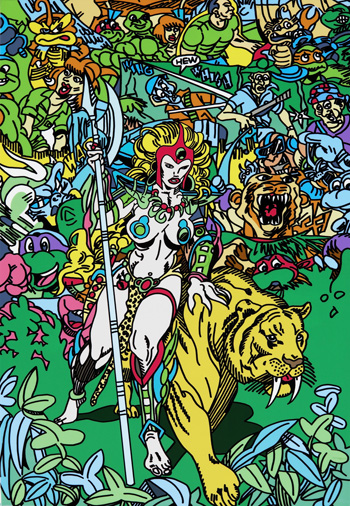The image is a colorful and vibrant graphical painting set against a predominantly light green background, depicting a jungle-like scene filled with various cartoon characters. At the center of the image is a white woman with blonde hair, adorned with a red headpiece. She is nearly nude, with bright blue rings covering her breasts and a few colorful chains around her body. She is wielding a large spear with a sword-like blade and is accompanied by a yellow tiger with black stripes and prominent saber teeth, which she is partially riding.

Surrounding the central figures are several characters and elements that contribute to a busy and dynamic scene. To the left is one of the Teenage Mutant Ninja Turtles wearing a purple bandana, and above him is a blue creature with a green helmet marked by a "V." Above them is April O'Neil from the Teenage Mutant Ninja Turtles, with another turtle beside her. Further up, there are two more turtles; one has a red bandana, while the other has none.

The right side of the image features another tiger with its mouth open and several additional characters, including a man in a green shirt, a worm-like creature, pirates, and more Ninja Turtles, identified by their red and orange bandanas. The entire scene is outlined in black, with bold, neon, and bright colors, creating a lively and striking visual composition.